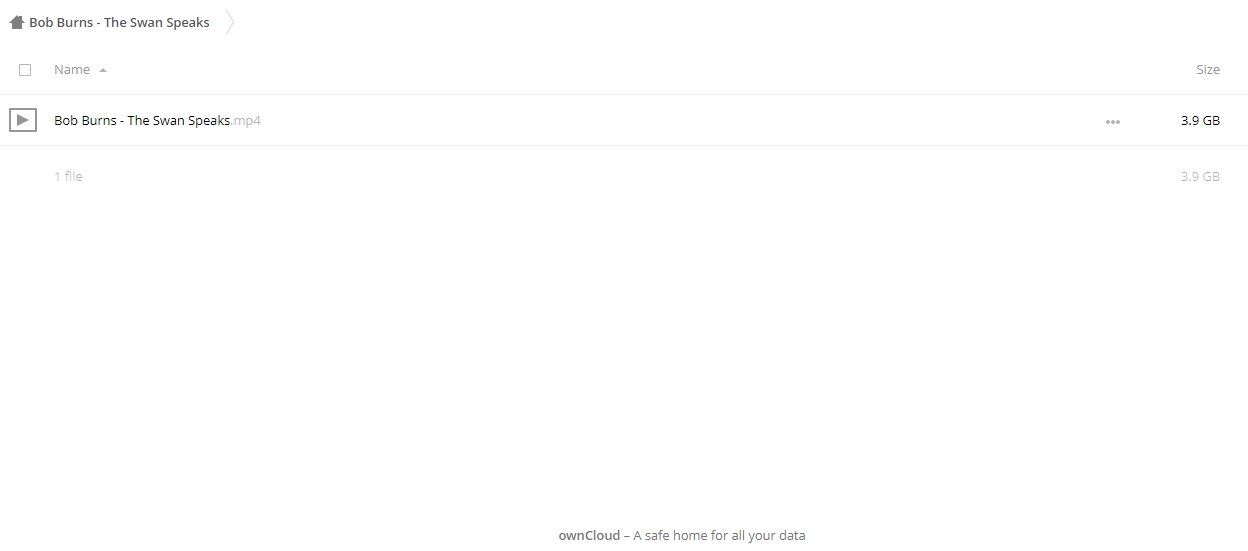Screenshot of a web page titled "Bob Burns - The Swan Speaks." At the top left, there is a home icon or arrow. Below the title, there is a gray area with the label "Name" next to an empty text box. Adjacent to this, in the next column, the text "Bob Burns - The Swan Speaks" appears prominently alongside a small rectangular play button with an arrow, indicating that this passage is an audio or video file. The file is identified as an MP4 format, with a size of 3.9 gigabytes, and there is one file available. At the bottom of the screenshot, there is a brand logo for "ownCloud - A safer home for all your data," suggesting that the MP4 file is stored on this cloud service for future access.